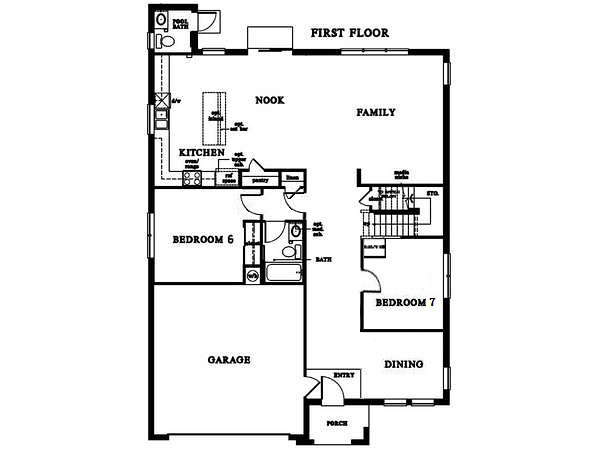This detailed black and white floor plan features a layout with a black background, black room outlines, and black text. It depicts the first floor of the building with key areas clearly marked. 

Starting from the bottom left corner, the garage is situated there, and to its right is the porch. Both the garage and porch provide entry points into the house, leading directly into the dining room. Adjacent to the dining room on the right is "Bedroom 7," which raises questions about the total number of bedrooms in the house or possibly the layout of the building.

Moving upwards from the dining room, a staircase is positioned, although this floor plan only showcases the first floor. To the left of the staircase, there is a bathroom equipped with a shower. Next to this bathroom lies "Bedroom 6," which notably includes two closets.

Progressing through the floor plan, to the right of this area is the family room. Additionally, there is a cozy nook adjoining the family room which leads into the kitchen. Completing the layout, a pool bathroom is located straight ahead, adding a convenient feature for this residence.